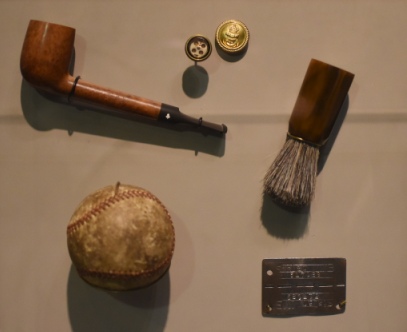The image features a display of six antique objects arranged on a whitish-brown background, possibly within a museum or a collection. Starting from the upper left-hand corner, there is a wooden pipe, indicative of traditional smoking habits. Directly below the pipe, situated in the lower left-hand corner, lies an old, well-worn baseball, exhibiting a brownish hue from age. Moving to the upper right-hand corner, a shoeshine brush is positioned, its bristles splayed out. In the middle, at the top, there is a decorative metal button or pin, though the specific design on it is unclear. The lower right-hand corner features a dark plaque or label, potentially made of copper or tin, with indiscernible etched text. The lighting in the photograph is coming from above, contributing to the low resolution and yellow tone of the image while casting shadows that emphasize the vintage and well-preserved nature of the artifacts.